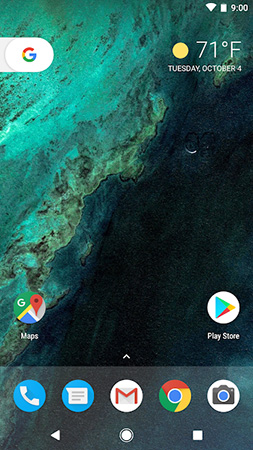This image displays an Android smartphone home screen with various app icons and interface elements. At the top-right corner, the status bar indicates the time is 9:00, alongside icons for Wi-Fi connectivity, battery status, and a temperature reading of 71 degrees Fahrenheit. The date is noted as Tuesday, October 4th.

Prominently featured app icons include Google Maps, the Play Store, a phone dialer, a text messaging app, Gmail, Google Chrome, and a camera preview. At the bottom, the familiar Android navigation button is visible for accessing the app drawer or home functions.

The background image is a top-down view of a vast expanse of water with minor rocky sections, giving a serene and expansive feel to the home screen. The overall setup is straightforward, showcasing a typical arrangement of essential apps and widgets for easy access.